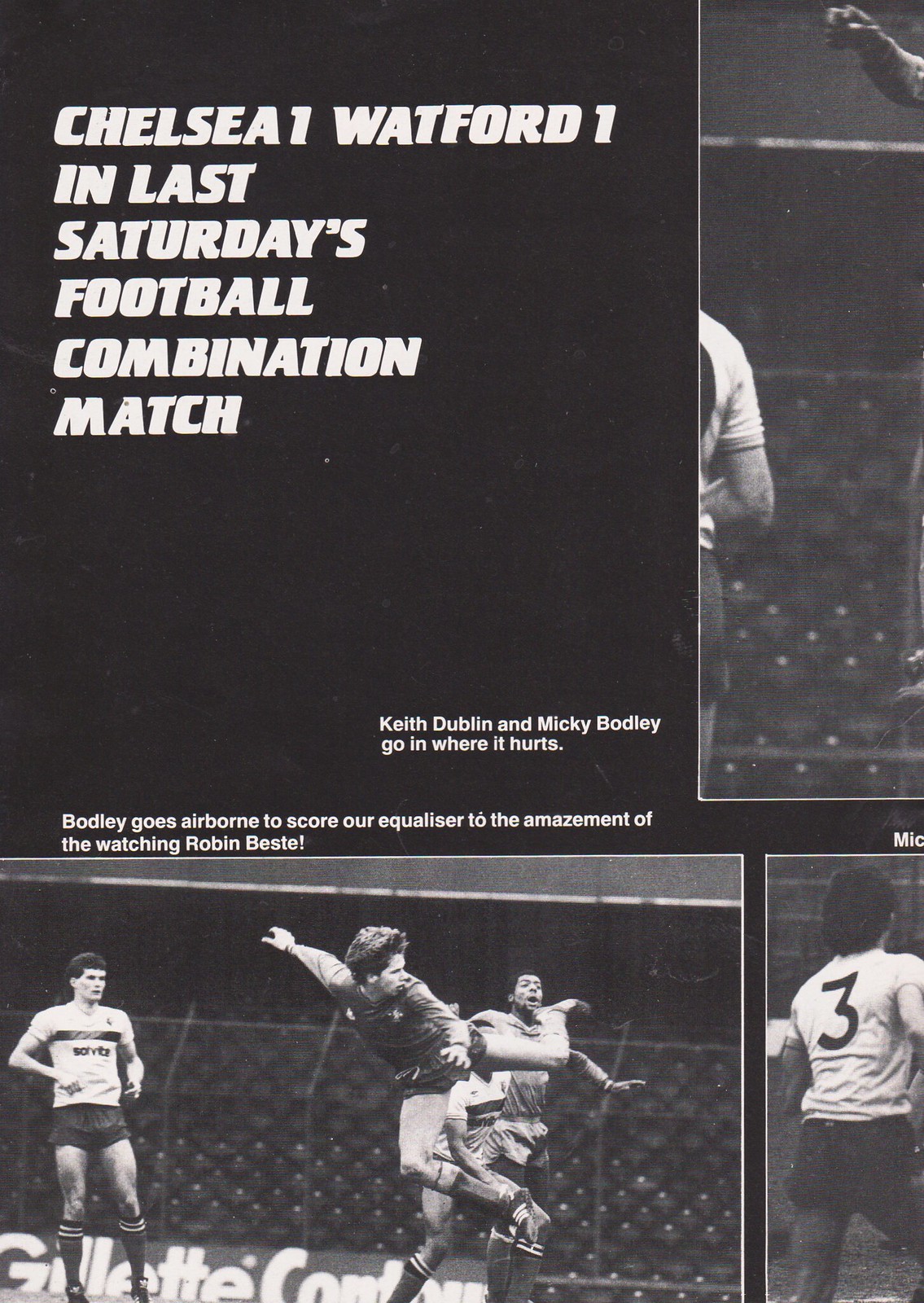This black and white image appears to be a page from a magazine or an advertisement displaying moments from a football match. The title at the top left corner reads, "Chelsea 1, Watford 1, in last Saturday's football combination match." The main caption underneath adds, "Keith Dublin and Mickey Bodley go in where it hurts. Bodley goes airborne to score our equalizer to the amazement of the watching Robin Best." The image contains multiple photos, though some are partially obscured. In one photo, a dramatic moment is captured where a player appears to perform a spinning kick, while another player watches on. Another visible image shows a man from behind, wearing a white shirt emblazoned with the number three. The players are dressed in typical football attire, including shorts, high socks, and cleats, highlighting the physical action and intensity of the match.